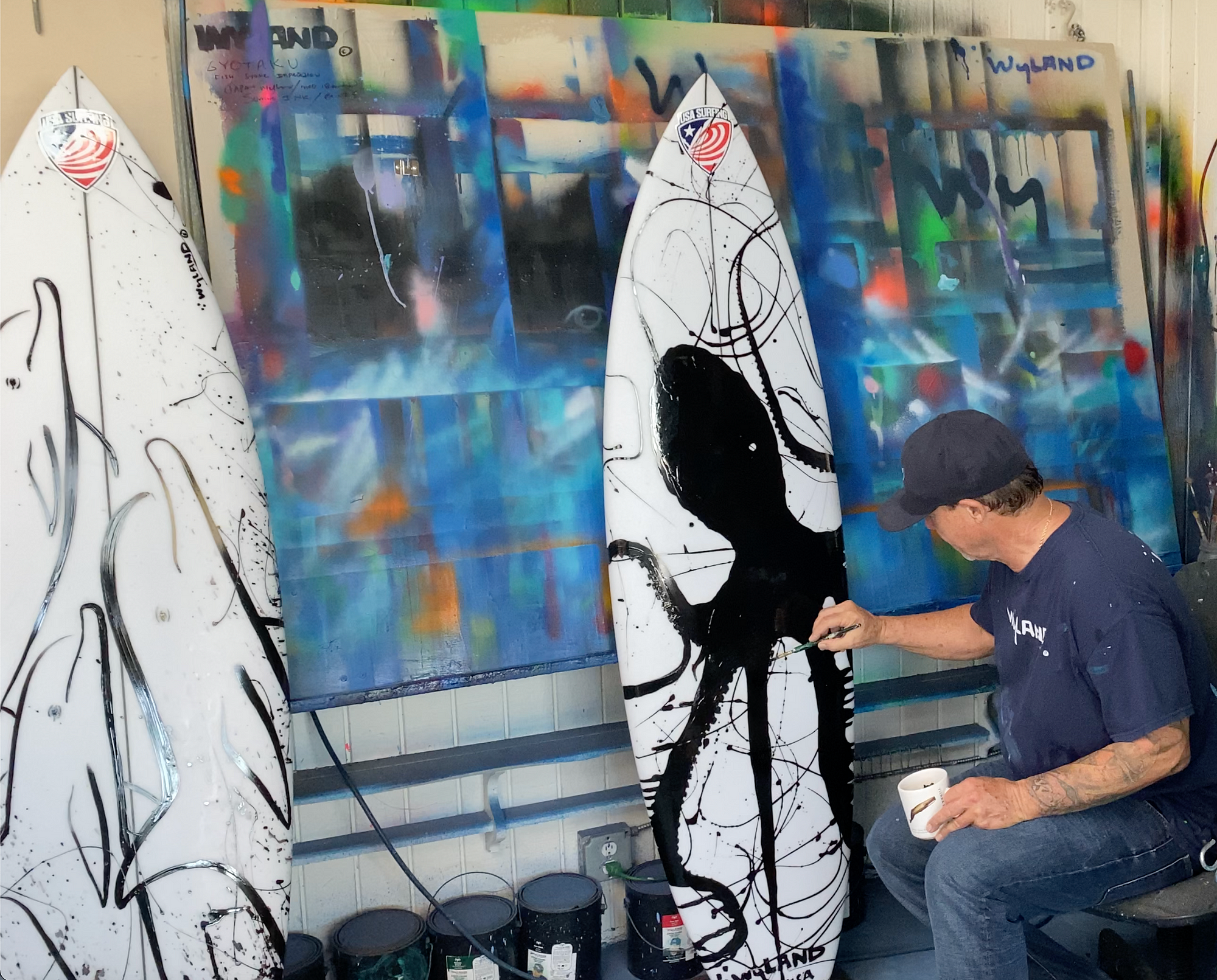In this detailed and artistic photograph, a middle-aged male artist is engrossed in painting a surfboard, showcasing his creative process. He sports a black cap, a dark blue t-shirt with white writing, and blue jeans. Seated at his workbench, he holds a small white cup of black paint in his left hand and a wide-brushed paintbrush in his right. Skillfully, he is painting a giant black octopus—described by others as squid-like—onto the pristine white surfboard, which bears the brand logo "U.S.A. Surfing" resembling an American flag. Next to him, a second surfboard leans against the wall, drying with a completed design of black lines meandering across its surface. Surrounding his workspace are several buckets of paint, and to protect his walls from accidental splatters, a paint-splattered board rests against the wall. In the backdrop, large, colorful spray-painted artworks add an additional layer of artistic atmosphere to the scene, capturing the essence of a dedicated artist at work.